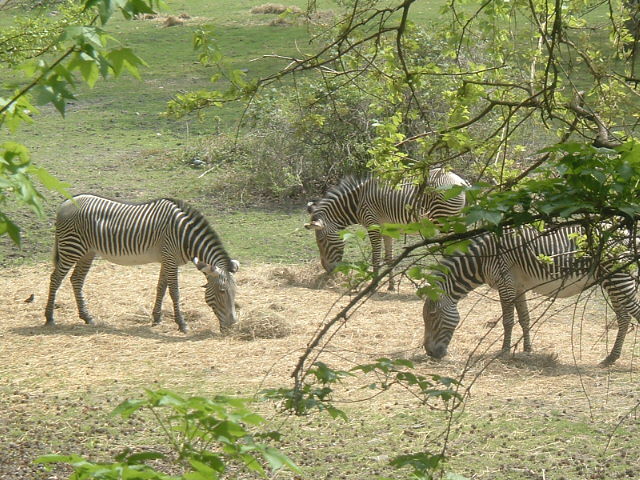In this image, three zebras with striking black and white stripes graze peacefully on a field of tan, straw-like hay. Their heads are bent down to the ground, engrossed in eating. The zebras are positioned in the middle of the image with varying orientations: two face left while one faces right. The dry hay they are grazing on extends halfway up the image, after which the terrain transitions into a thin layer of green grass that seems to slope upward, forming a gentle hill. Surrounding the zebras is lush foliage with vivid green leaves hanging from tree branches descending from the top left and right corners, and there's a smattering of smaller green plants near the bottom. The scene is set in a woodsy countryside, with the leafy branches creating a natural frame around the zebras. The green leaves and branches lend a three-dimensional effect to the scene. In the background, there are clusters of brush and a large bush beyond the zebras, and barely visible at the top left and right are piles of hay. The meticulously striped zebras feature a distinctive mane resembling a mohawk, made of dark gray fur, extending from between their ears down their necks. Shadows cast by the zebras add to the depth of the field. The serene setting is momentarily punctuated by a small bird on the ground to the left of the zebras.